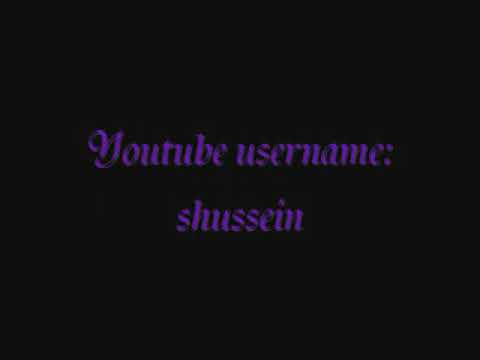The image features a gradient background transitioning from dark orange at the top and bottom to a lighter, richer orange in the center. At the top of the image, there are two lines of text in Arabic, written in white. Beneath the Arabic text, there is an English translation that reads, "Bless Muhammad and the household of Muhammad." This English text is also in white and written in a simple font, placed in the middle to bottom part of the image. The Arabic and English texts together dominate the image, which has no borders, allowing the vibrant orange gradient to fill the entire space.